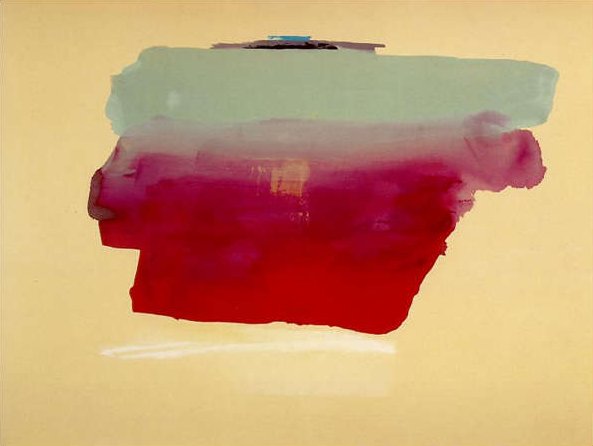This image features an abstract painting titled "Robinson's Rap" by Helen Frankenthaler, created in 1974. The canvas is oriented in landscape and has a yellowish-orange, beige background. The composition is predominantly defined by horizontal color blocks. Near the top, a thick, seafoam green horizontal stripe runs across, slightly blending with the underlying colors. Below this stripe lies a wide red rectangle that transitions to a pinkish hue, adding depth to the artwork. This red area appears as wet-looking horizontal stripes. Interspersed within the red are light white horizontal strokes near the bottom. Near the center, a lightly shaded yellow square gives an impression of a lock, evoking the imagery of a trunk. A thin dark blue horizontal stripe rests above the seafoam green area. The overall style is color blocking with an abstract presentation, typical of modern art.